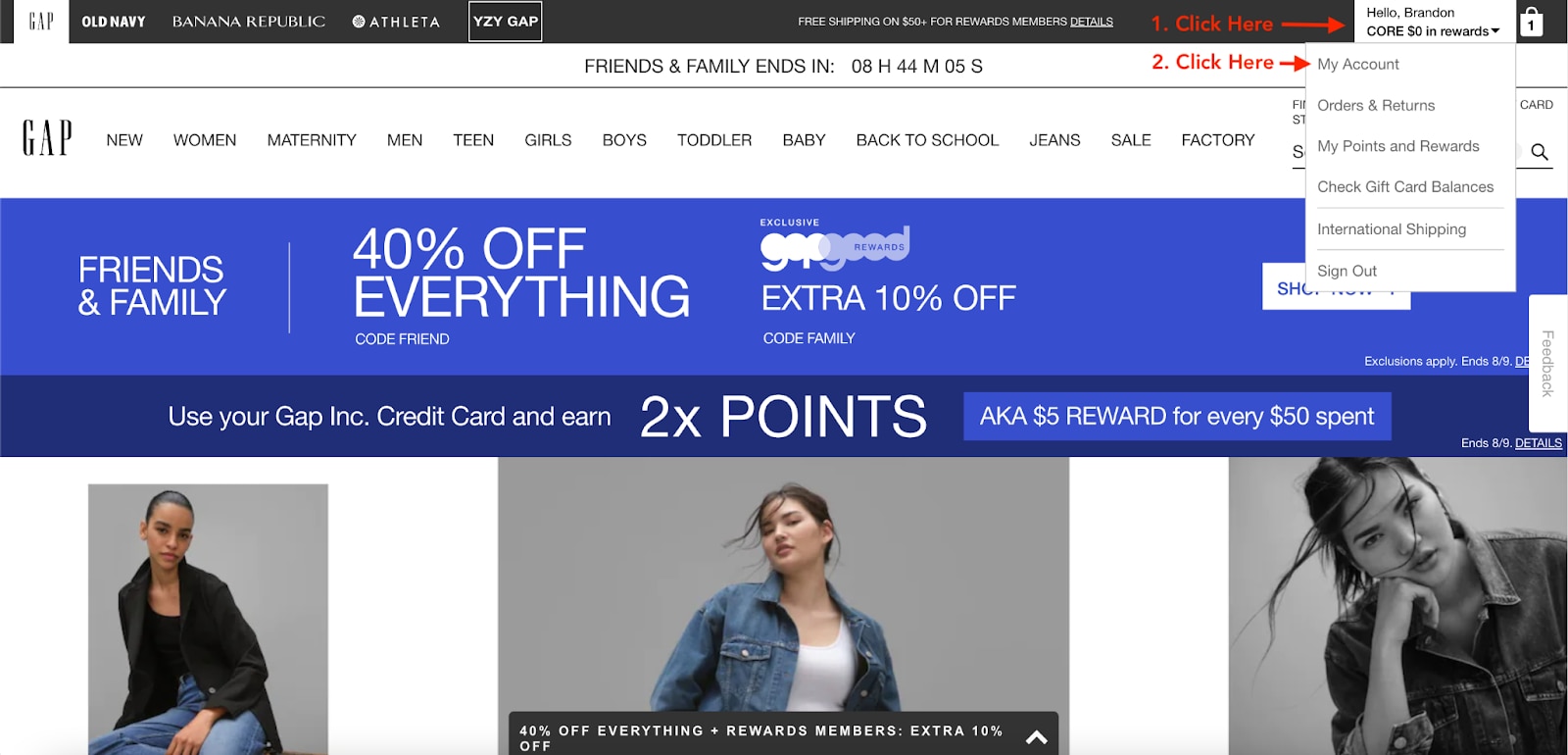A detailed descriptive caption for the image could be:

"A screenshot of the top section of the Old Navy landing page, guiding users on how to log in to their accounts. The top-right corner features a 'Log In' button and a personalized greeting, 'Hello Brandon,' both highlighted prominently. Nearby, a red label marked with the number '2' emphasizes the 'My Account' dropdown menu. Beneath the navigation bar, a blue promotional banner announces '40% off everything,' part of the site-wide Friends and Family sale. The banner is complemented by images of smiling girls wearing stylish denim jackets, illustrating the current fashion offerings. The overall layout focuses on the login process while showcasing Old Navy's latest deals and trendy apparel."